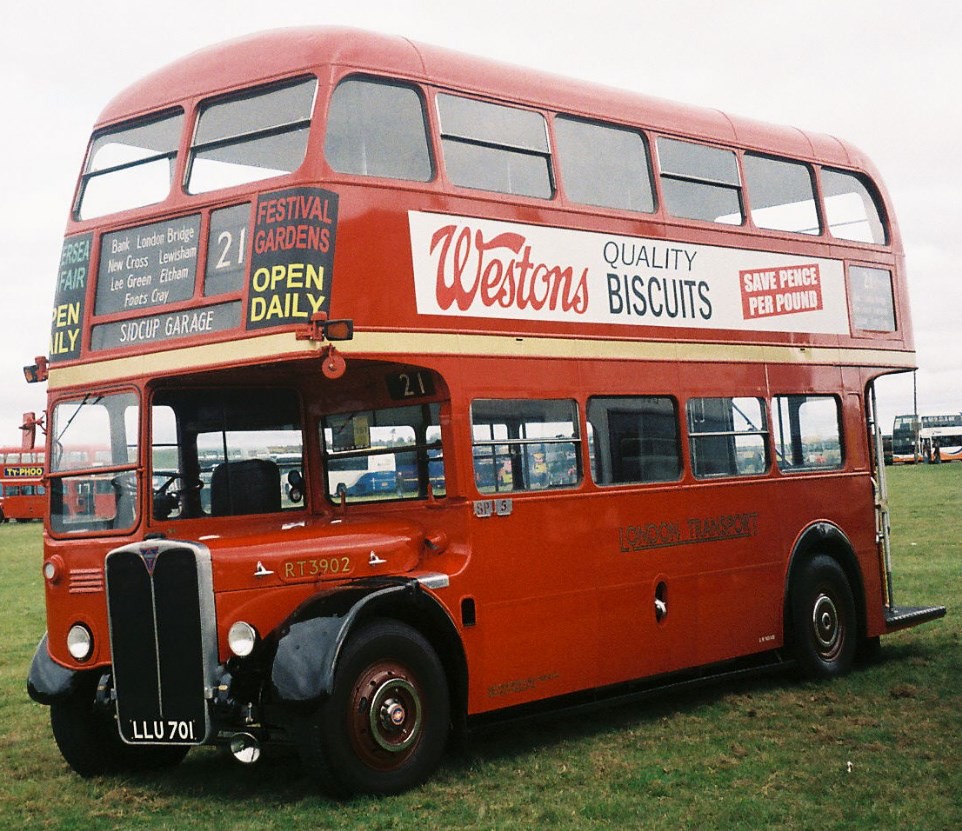This is a wide rectangular photograph of a historic red London double-decker bus, prominently tilted diagonally with the front on the left side, closer to the camera than the back. The bus, possibly exhibited in an open field reminiscent of a museum piece, is parked on neatly trimmed green grass. The sky is overcast with grey clouds, typical of England. 

The bus features numerous advertisements: prominently displayed between the upper and lower windows is a white rectangular sign with "Westin's" in red fancy font, followed by "Quality Biscuits" in black letters, and a tilted red rectangle with "Save Pence Per Pound" in white font. The front of the bus bears the route numbers and destinations, stating "Bank London Bridge, New Cross, Lewisham, Lee Green, FM, Footscray, Sidcup Garage," and the route number "21." Below, a gold inscription reads "London Transport," which is also repeated in black letters at the bottom of the lower half. 

Additional details include the bus number "RT3902" on the side and the license plate "LLU701." Surrounding the main bus in the background are old cars, hinting at the setting being an antique car show. In the distance to the left, another red bus can be seen. No people are visible in or around the bus, adding to the timeless quality of the scene.